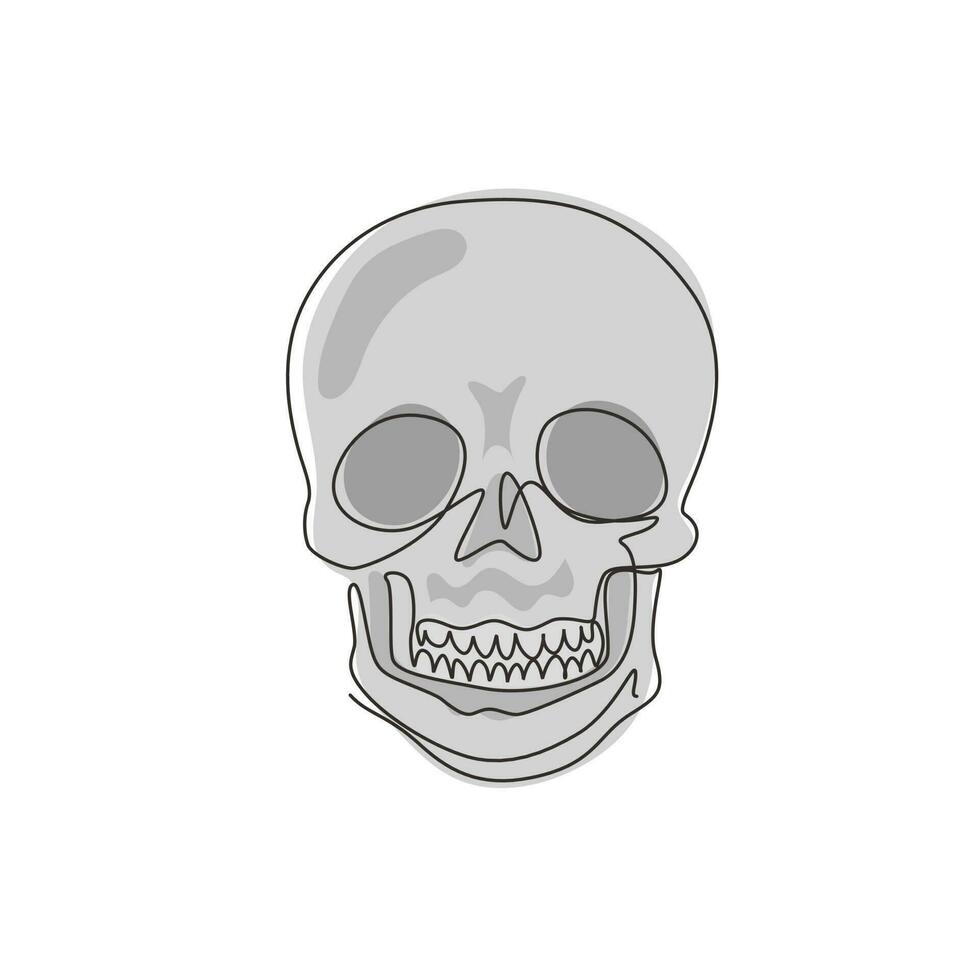This image is a hand-drawn sketch of a human skull, centrally positioned with no background or text. The skull is bordered by a black outline, emphasizing the jaw, teeth, nasal cavity, and eye sockets. The entire skull is filled with varying shades of gray: the lighter grays dominate the overall face and teeth, while darker grays accentuate the eye sockets, nasal cavity, and certain facial features like the chin and brow. The depiction of the teeth is uneven and wavy, suggestive of a cartoonish style rather than a realistic approach. The top of the skull and areas under the nose and chin are rendered in darker grays, adding some depth and shading to the image. Despite these details, the drawing lacks intricacy and has a simplistic, hand-drawn quality, characterized by its cartoon-like appearance.